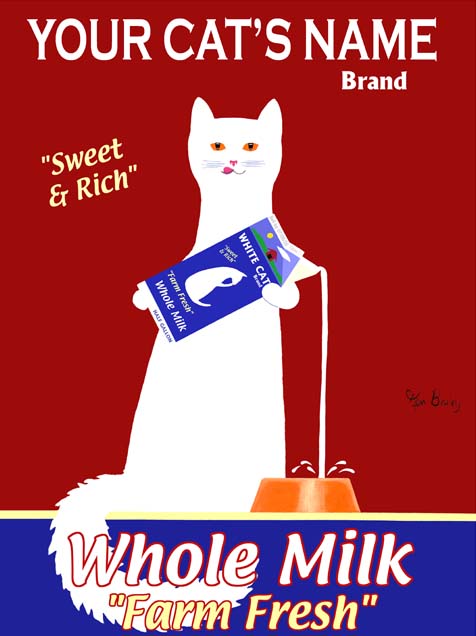This illustration exudes the charm of a vintage silkscreen poster, featuring a white cartoon cat with a playful expression. The cat, standing upright and resembling a human, prominently displays its vibrant yellow eyes and a pink tongue peeking out as if licking its lips. Against a striking cherry red background, the feline pours milk from a carton labeled, "White Cat Farm Fresh Whole Milk," into an orange cat bowl at its feet. The words "sweet and rich" accompany the scene in quotations to the left side of the cat. 

At the top, the customizable banner reads, "Your Cat's Name" in bold letters followed by "Brand," suggesting the ability to personalize the poster with any cat's name. Artistically, the poster also incorporates a blue rectangle at the bottom with a yellow stripe, showcasing the text, "Whole Milk Farm Fresh." The artist's signature in black adorns the right side, encapsulating the vintage allure of this whimsical and delightful milk advertisement.